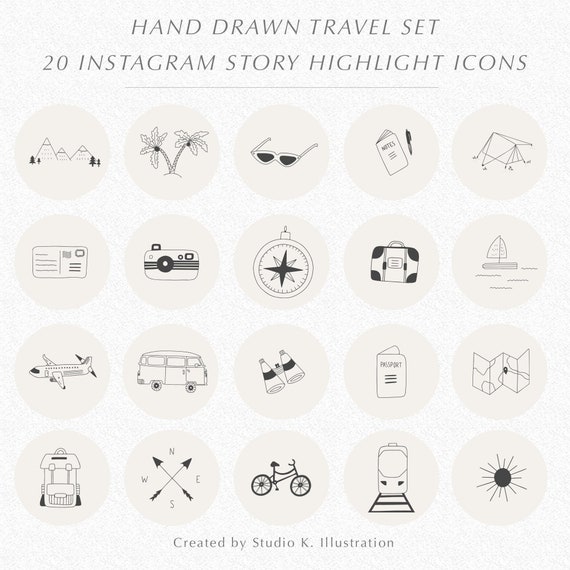This image is an advertisement for a "Hand-Drawn Travel Set" featuring 20 Instagram story highlight icons, and is created by Studio K Illustrations. The illustration organizes these black-and-white travel-themed icons over cream-colored circular backgrounds, arranged across four rows from left to right. Starting at the top, the icons depict: a mountain with trees, palm trees, a pair of sunglasses, a travel itinerary or notebook with a pen, and a tent. The second row features a postcard or travel pass, a camera, a compass, a suitcase, and a sailboat. Continuing to the third row, there is an airplane, a van, binoculars, a passport, and a map. The final row includes a backpack, a compass rose, a bicycle, a train, and a sun. These simple yet detailed illustrations are set amid a tan-colored background with light speckles, giving the overall design a cohesive and artistic feel.